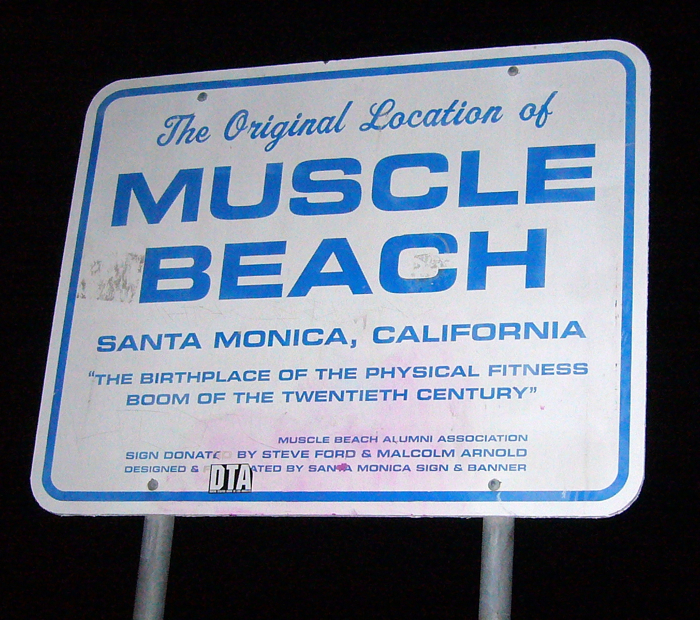The image captures a slightly worn and rusted metal sign at Muscle Beach in Santa Monica, California, illuminated by camera flash against a completely dark night sky. The sign, held up by two standard silver metal poles, features a white background with a thick blue border and various text fonts and sizes. The largest text, "Muscle Beach," is prominently displayed at the top in all capital letters, followed by "The original location of Muscle Beach" and "Santa Monica, California" in smaller fonts. Beneath this, a quotation reads, "The birthplace of the physical fitness boom of the 20th century." Lower down, the sign acknowledges the Muscle Beach Alumni Association and notes that it was donated by Steve Ford and Malcolm Arnold, with its design attributed to Santa Monica Sign and Banner. Additionally, there is a small black sticker with white letters at the bottom of the sign reading "DTA," alongside some signs of pink residue and other minor markings.